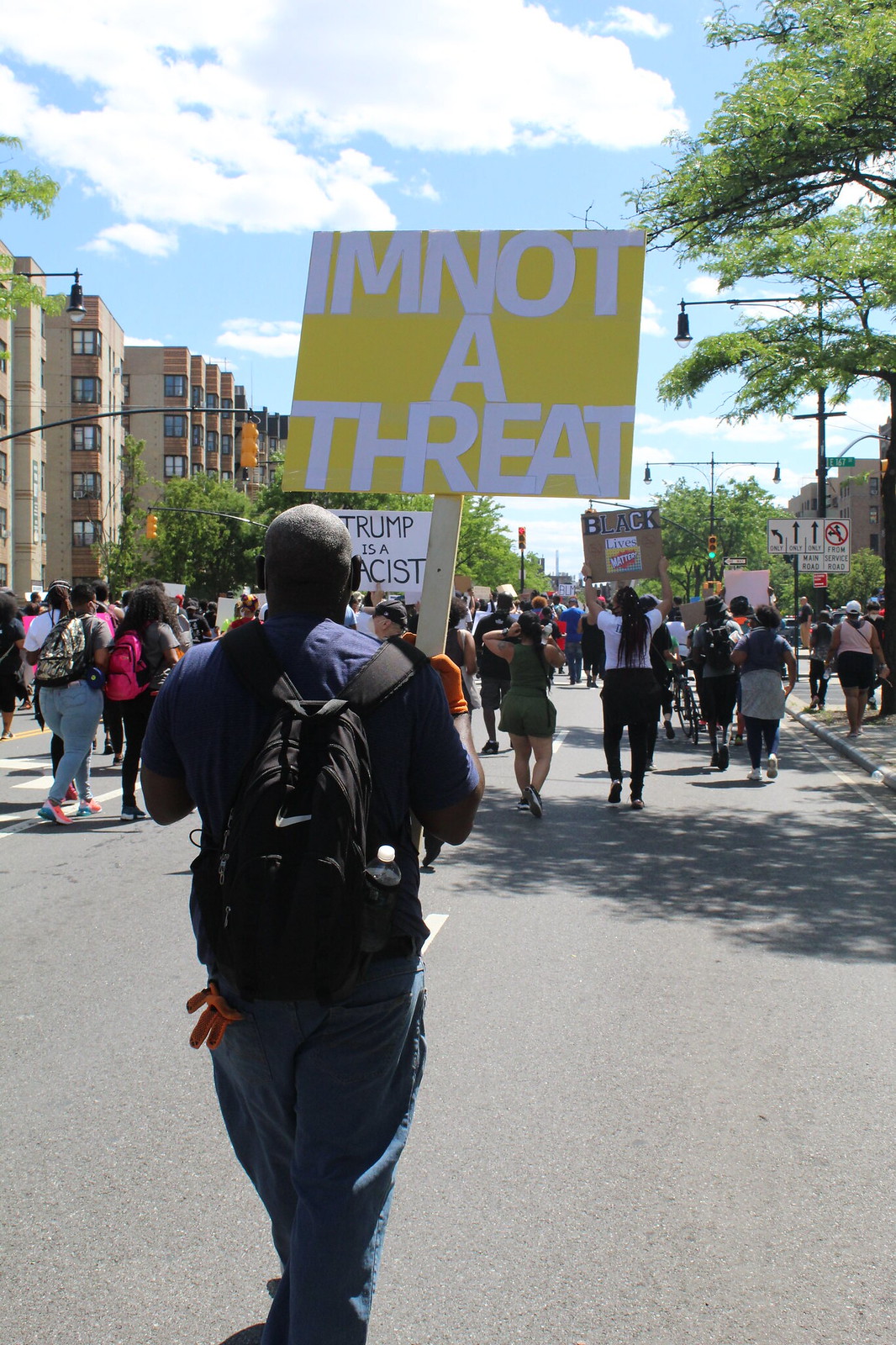A large crowd of protesters walks down a light gray asphalt street, partially shaded by the shadow of a tree in the bottom right corner. Dominating the center of the scene is a Black man slightly to the left, dressed in a blue shirt and carrying a black backpack. An orange glove dangles from one of his back pockets. Holding a wooden stick with a sign high above his head, it features a yellow square with bold white letters proclaiming, "I'm not a threat." 

Spread across the width of the street, various other protesters can be seen. To the right, a woman with dark black hair, dressed in a white shirt and black pants, holds a cardboard square above her head that displays the word "Black." On the left, another protester lifts a white sign bearing black letters, partially visible with the text "Trump is a racist," with only "C-I-S-T" clearly readable.

Framing the left side of the image are tall, light cream-colored buildings that resemble a hotel. Traffic lights, suspended from bars, extend into the scene from both sides. The upper left section of the image shows the tips of some tree branches with green leaves, while more prominent branches with thick foliage extend from the right side. The sky in the background is a mix of light blue with scattered white and gray clouds, adding to the vivid atmosphere of the protest.